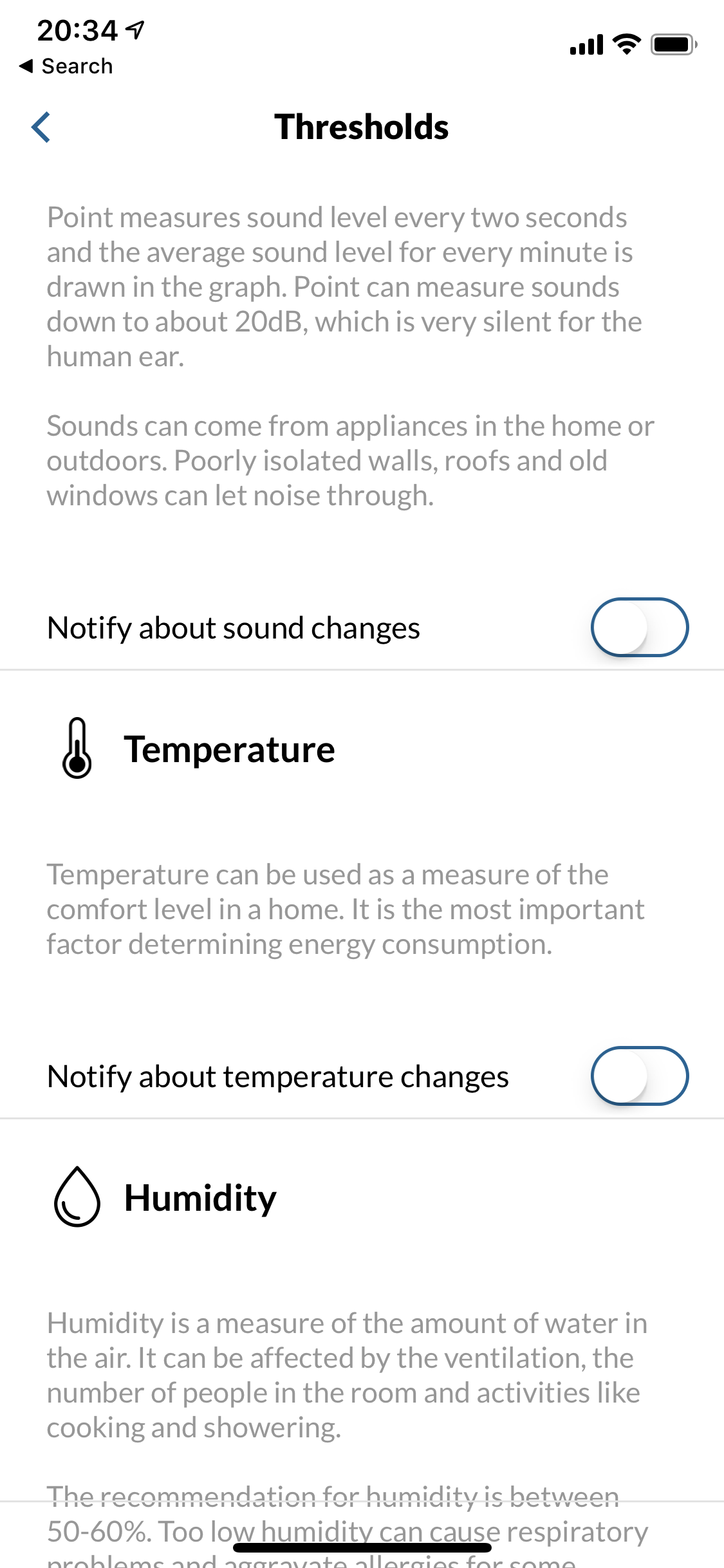In the image, a phone display showcases an application screen dedicated to monitoring environmental conditions such as sound, temperature, and humidity. At the top right corner, the status bar indicates a strong Wi-Fi signal with five bars and a fully charged battery. The time displayed is 20:34, or 8:34 PM, and the word "search" is visible on the left side of the screen.

The primary focus is on three key metrics: sound, temperature, and humidity. Under the "Sound" section, the app description explains that it measures the sound level every two seconds and calculates the average sound level per minute, which is graphically represented. It notes that the measurement sensitivity can go as low as 20 decibels, which is nearly imperceptible to the human ear. It also mentions how household appliances, outdoor noises, poorly insulated walls, roofs, and old windows can contribute to ambient sound levels. There's an alert option to notify users about changes in sound levels, currently toggled off.

The next section, labeled "Temperature," includes a bold heading with a thermometer icon. It discusses how temperature is crucial for assessing comfort levels in a home and is a significant factor in energy consumption. Similar to the sound section, there is a notification option for temperature changes, which is also turned off.

The final section, "Humidity," describes it as a measure of the water content in the air and explains its dependency on ventilation, the number of people in the room, and activities like cooking and showering. The recommended humidity range is stated to be between 50 to 60%, with too low humidity potentially causing respiratory problems and aggravating allergies. The text at the bottom is cut off, and a partial view of the phone's bottom edge is visible.

Overall, the display is an informative and detailed interface for tracking and managing home environment conditions.